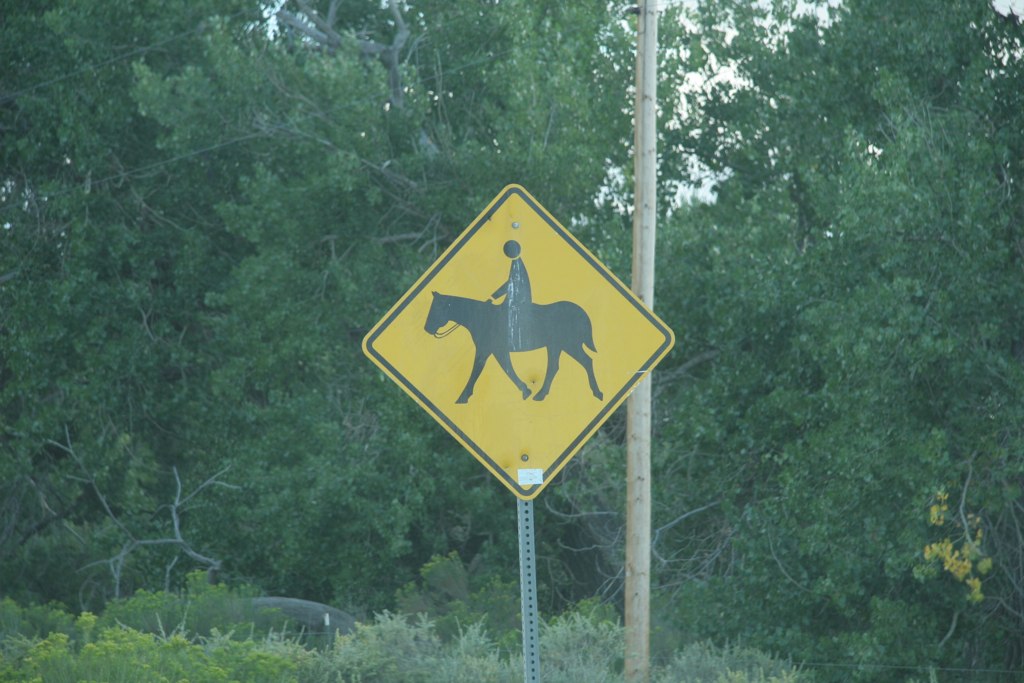This horizontal, rectangular photograph captures a dense forest scene with lush green trees and bushes, with a small patch of grayish sky peeking through. The image is somewhat blurry and out of focus, likely taken with a dirty lens. Front and center in the photograph is a yellow road sign with a black border and a depiction of a person in a filled-in black garment riding a horse. The sign is diamond-shaped, standing upright on one of its corners, and mounted on a slender, gray metal pole with several dots running down its length. A small white sticker is visible at the bottom center of the sign. To the right of this road sign is a utility pole with visible cables extending towards the upper left of the image. Sunlight breaks through the trees slightly, adding a touch of light to the dense foliage that forms the backdrop.